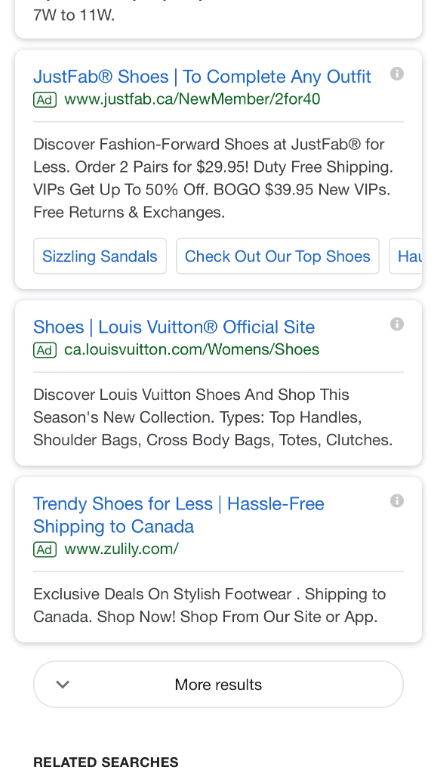This is an image of a cell phone screen displaying a selection of online shopping links for shoes. At the top, the partially visible link mentions shoe sizes ranging from 7W to 11W. Below, there's a prominent ad for JustFab, which includes the text: "JustFab shoes to complete any outfit." The link provided in the ad is www.justfab.ca/newmember/2for40. The advertisement touts their offerings: "Discover fashion-forward shoes at JustFab for less. Order two pairs for $29.95! Duty-free shipping. VIPs get up to 50% off. BOGO $39.95. New VIPs: Free returns and exchanges." There are clickable buttons for "Sizzling Sandals" and "Check Out Our Top Shoes," though the last button's text is cut off. The next listing showcases "Shoes - Louis Vuitton Official Site," identified as an ad, inviting users to "Discover Louis Vuitton shoes and shop this season's new collection," with categories including top handle, shoulder bags, crossbody bags, totes, and clutches. Additionally, another listing promotes “Trendy Shoes for Less” with the benefit of "hassle-free shipping to Canada."